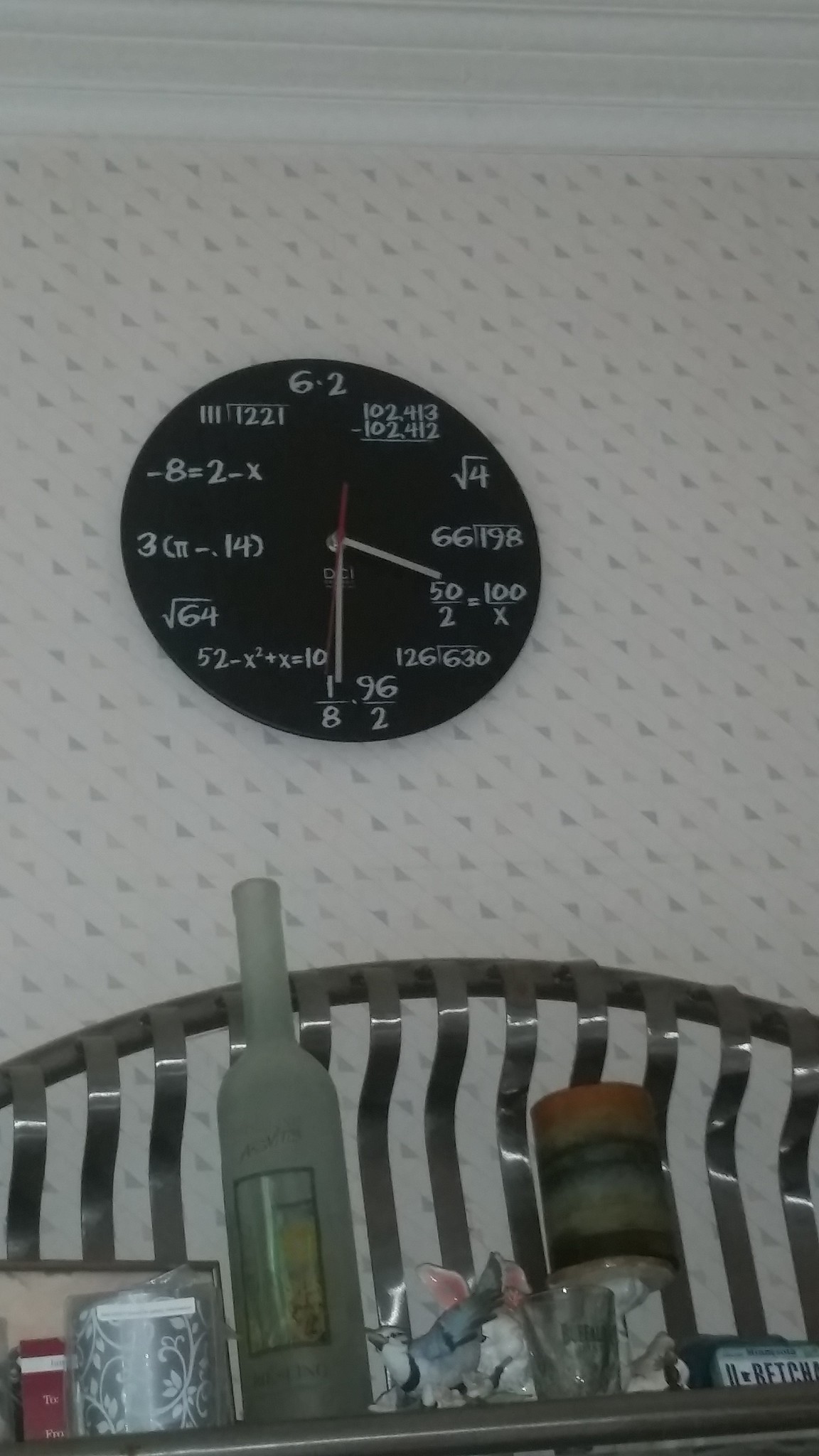This image features a unique clock prominently displayed on a white wall adorned with subtle gray dots. Positioned slightly off-center toward the left, the clock stands out with its black face and contrasting white clock hands. Adding a clever twist to standard time-telling, the clock face replaces traditional hour numerals with mathematical equations whose solutions correspond to the respective hours. For instance, the 12 o'clock position features the equation "6 x 2," symbolizing 12. 

Beneath the clock, a table or stand serves as a small bar area, cluttered with an assortment of items. Among the items are a candle, several shot glasses, various bottles of alcohol, what appears to be a pack of cigarettes, and framed photo. The overall setting merges the intellectual curiosity sparked by the math-themed clock with the casual, eclectic vibe conveyed by the objects below.